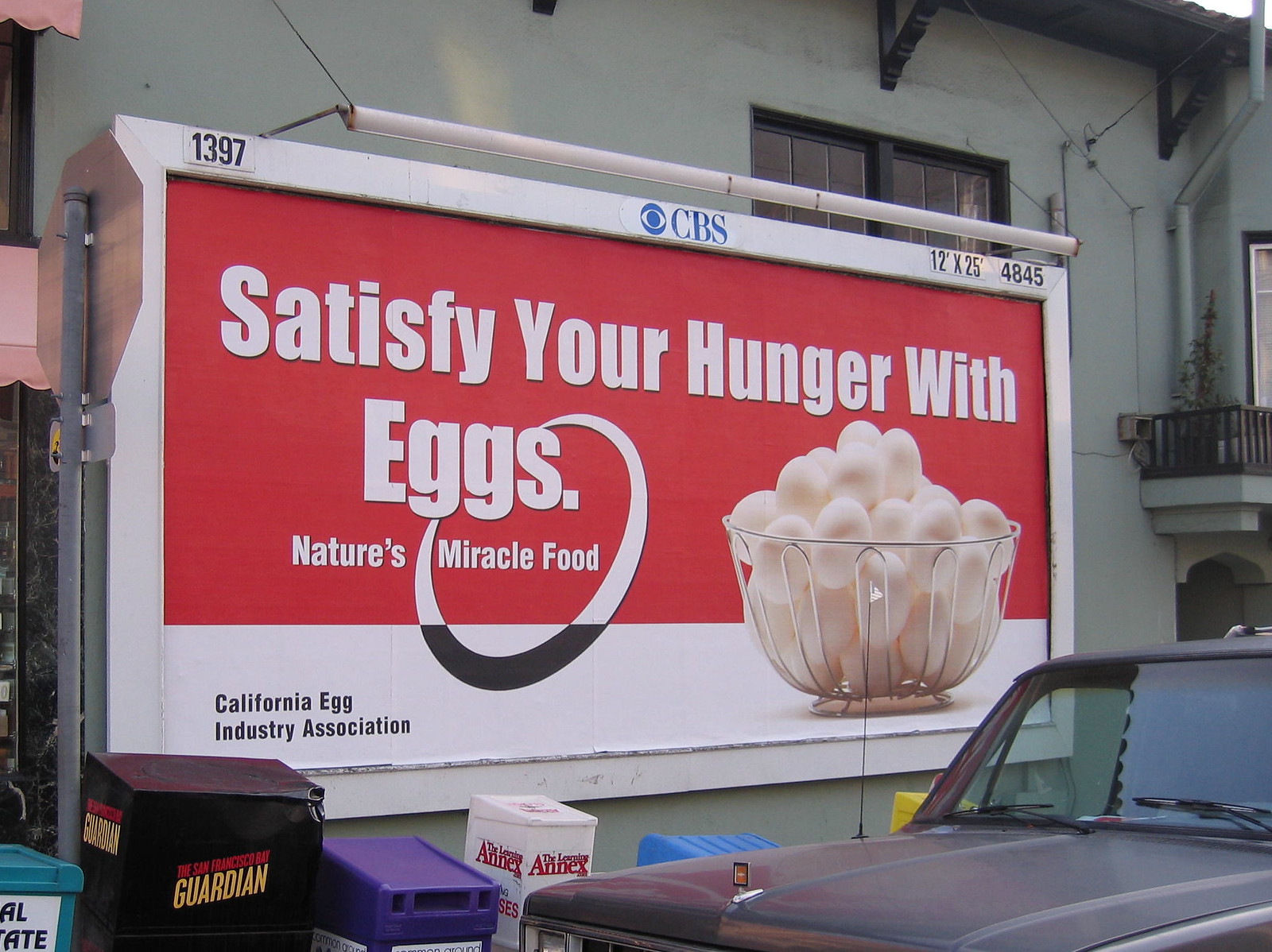A large, vibrant billboard is prominently displayed, either attached to or very near a pale greenish-gray building with windows, possibly indicating an apartment complex or another residential structure. The billboard, set against a red background with white text, reads, "Satisfy your hunger with eggs, nature's miracle food" and is an advertisement from the California Egg Industry Association. It also mentions "big red ringtone" and underscores the health benefits with "100% eggs." The prominent CBS symbol, in blue and white, is located on the top left, and there are alphanumeric designations "1397" and "12 by 25, 4845" spread across different areas of the billboard, suggesting dimensions and perhaps publication details from CBS Advertising. To the right of the billboard is a wired silver basket filled with white eggs.

In the foreground, a vintage gray car, likely from the 1970s, is parked, giving a glimpse of its old-timey windshield and a visible antenna on its roof. The street scene includes various newspaper vending machines from The Guardian and recycling bins. There is also a stop sign with the metal back facing us. The setting feels urban, with the hint of railings on the far right and newspaper sections lying scattered around. The overall layout suggests a busy street corner, bringing attention to both vehicular and pedestrian elements in the image.